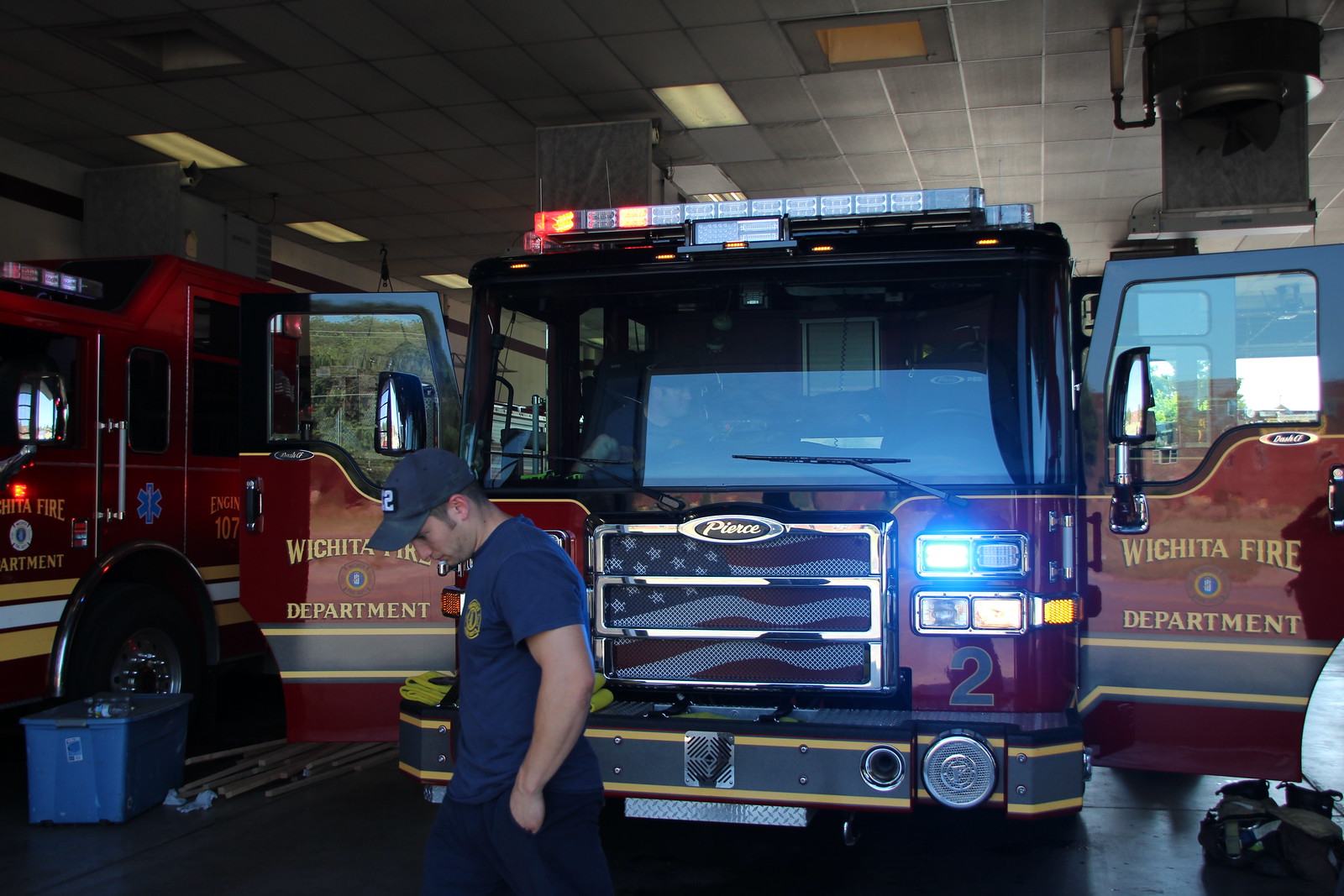The image depicts an indoor scene at a fire station garage, featuring two fire trucks. The focal point is a striking red fire truck in the center with both its front doors open, displaying the yellow lettering "Wichita Fire Department." The truck is embellished with a silver grille showcasing an American flag design, distinguishing it from typical vehicles. Below the right headlight is a gray number "2," and the bumper is gray with white borders. Positioned beside the truck is a man of Caucasian descent, wearing a blue ball cap, short-sleeved blue shirt with a fireman's emblem on the chest, and blue pants. He is depicted with his hands in his pockets, head tilted downward, and a cigarette in his mouth. The garage is dimly lit by recessed fluorescent lighting in a paneled ceiling, capturing a somewhat dark and enclosed atmosphere. To the left, a portion of another red fire truck is visible with the text partially obscured, adding to the overall setting of readiness and activity at the fire station.